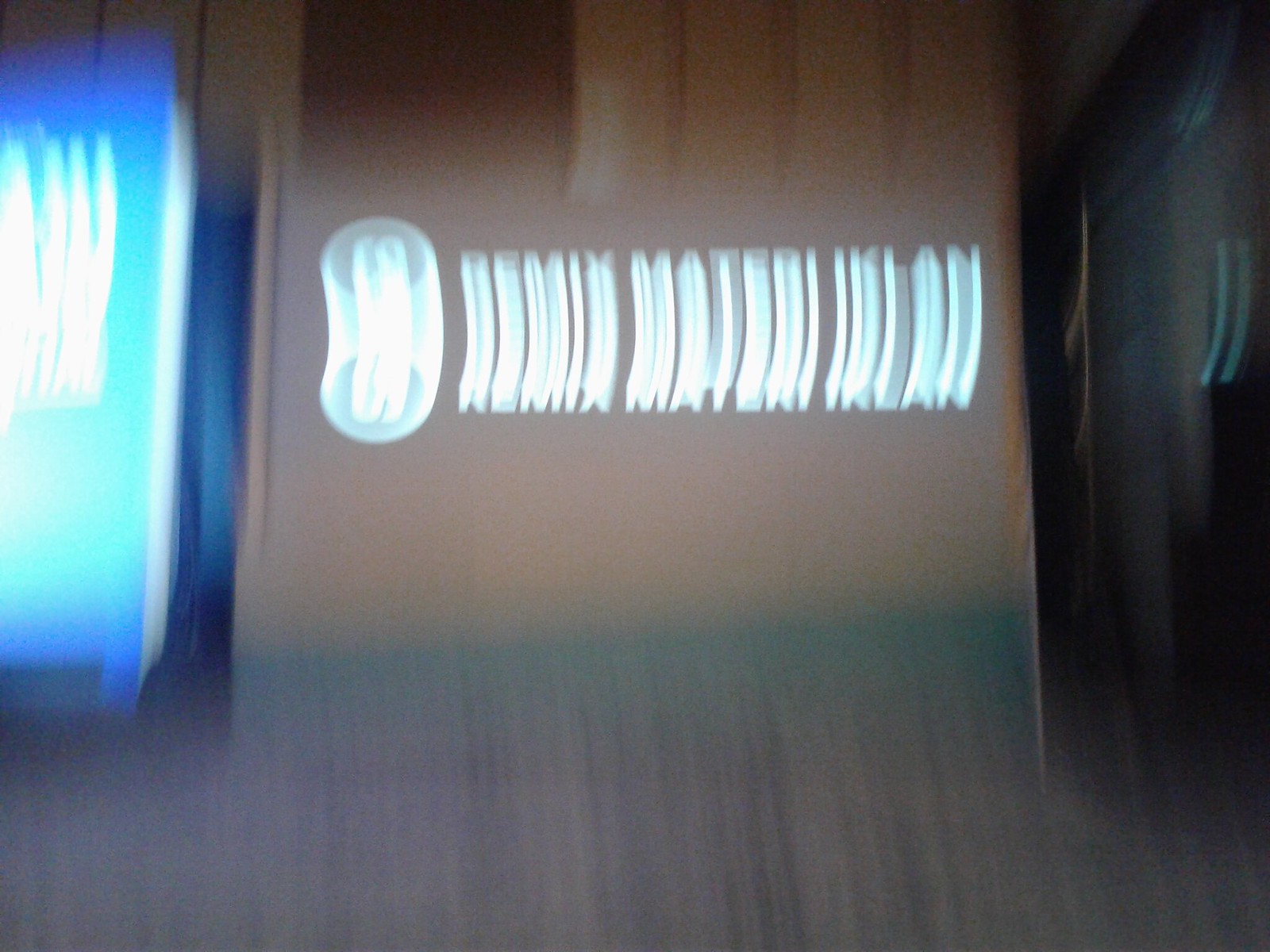This photograph appears to be quite blurry, making the details difficult to distinguish clearly. At the bottom of the image, the ground is a hazy gray with vertical lines disrupting the clarity. In the center, there is a section of a wall or possibly a poster set against a brown background. It features bright, shiny writing that includes a prominent oval shape. The text seems to be structured in segments: the first segment has five letters, followed by a space, then a segment with six letters, another space, and additional characters and spaces that are unreadable due to the blur. On the left side of the image, there is a blue area, likely another blurred sign. The overall lack of focus makes it challenging to discern more specific details about the scene.